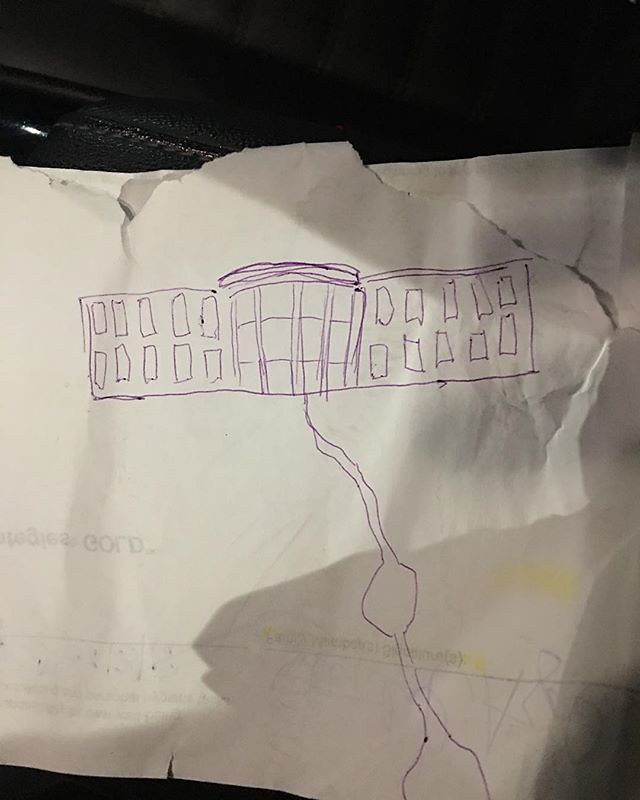This image depicts a crudely drawn depiction of what appears to be the White House in Washington, D.C., rendered in purple biro ink. The sketch is quickly executed, likely by an unskilled hand, and shows the iconic rounded design reminiscent of the Oval Office's exterior, complete with numerous windows. The drawing is on a white, tattered piece of paper with torn edges and prior writing, visible in reversed black letters, on the other side. A pathway extends from the building towards the bottom edge of the paper. Additionally, there are peculiar elements on the paper, such as a remote control-like rectangle with multiple buttons and some string-like lines with ball shapes. Notably, there are three small urine stains in the bottom right corner of the paper.